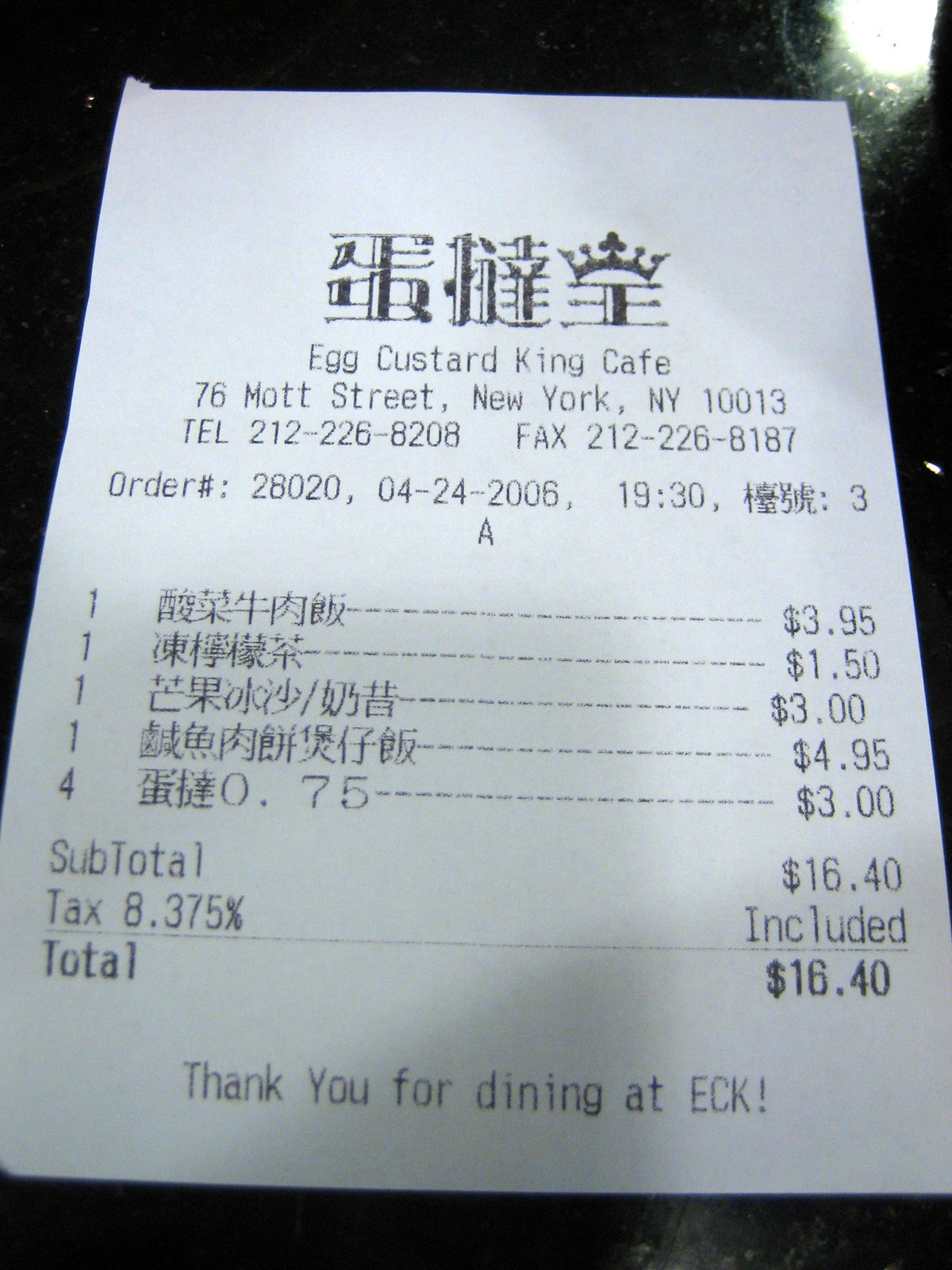This image is a receipt from the Egg Custard King Cafe, which was located at 76 Mott Street, New York, NY 10013. The top of the receipt features the company's logo with Chinese characters, including a crown on the final symbol. The receipt is printed on white paper with black text. Below the logo, it includes the cafe's phone number (212-226-8208) and fax number (212-226-6187).

The receipt is dated April 24, 2006, at 19:30, and has an order number of 28020. The list of ordered items appears in Chinese, with the respective prices: $3.95, $1.50, $3.00, $4.95, and $3.00, totaling $16.40, including tax. The bottom of the receipt concludes with a message, "Thank you for dining at ECK," indicating the abbreviation for Egg Custard King. The establishment has since closed down.